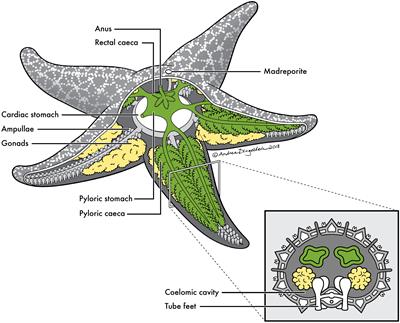This image is a detailed scientific diagram of a starfish, set against a white background. The central illustration features a gray starfish with its lower half depicted in a cross-section, revealing its interior anatomy. Various anatomical components are clearly labeled with black lines and text. These labels include prominent structures such as the anus, rectal coecum, madreporite, cardiac stomach, ampullae, gonads, pyloric stomach, and pyloric caeca.

The internal section reveals complex green frond-like structures resembling leaves and stems, along with tan-colored organs. Additionally, there is a yellowish substance, possibly representing internal body fluids or tissue, and spiky, bony structures forming the legs of the starfish. 

In the bottom right corner, a black rectangle with a gray background features an inset diagram showcasing a different perspective of the starfish's interior. This smaller diagram highlights the coelomic cavity and tube feet with additional black lines pointing to these specific parts.